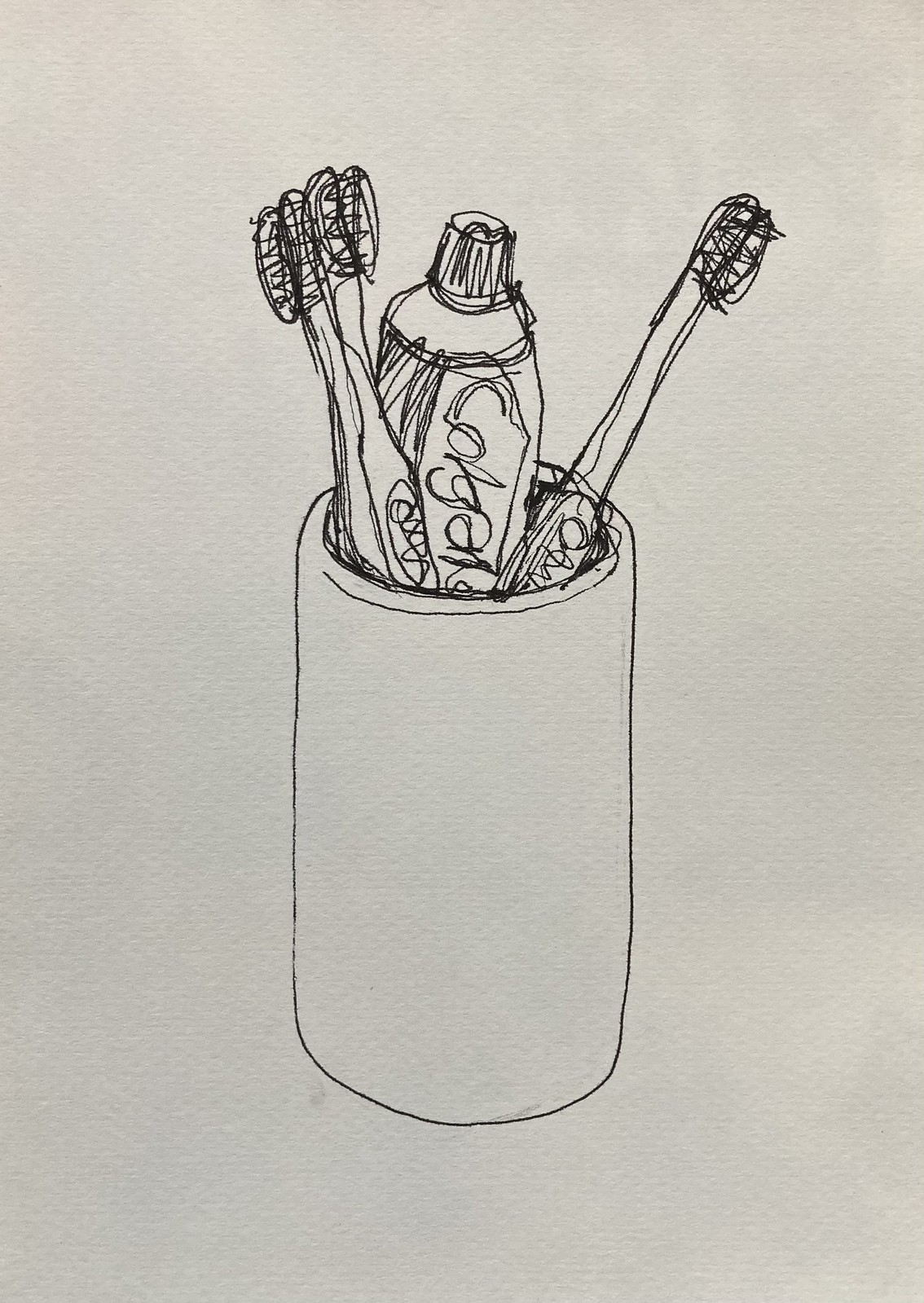In this detailed sketch, a tall, cylindrical container, resembling a can or a toothbrush holder, is filled to the brim with three toothbrushes and a tube of toothpaste, all standing upright and tightly packed together. The drawing is rendered in either black pen or thin black marker on a textured, off-white paper, which adds a subtle and artistic background to the image.

The toothbrushes, two positioned on the left and one on the right, have their bristles scribbled with upward strokes; the bristles on the left-most toothbrush are distinctively curved toward the left. Each toothbrush has an indiscernible label written along the handle. In the center of the container stands a tube of toothpaste with a cap illustrated using zigzag lines to depict grip ridges. Though the text on the tube is not fully clear, partial letters are visible, suggesting the brand name "Colgate."

The overall composition of the sketch places the container prominently in the center, with each object meticulously detailed despite their tight fit within the holder. This drawing, with no identified author, captures a simple yet intricate representation of everyday bathroom essentials.